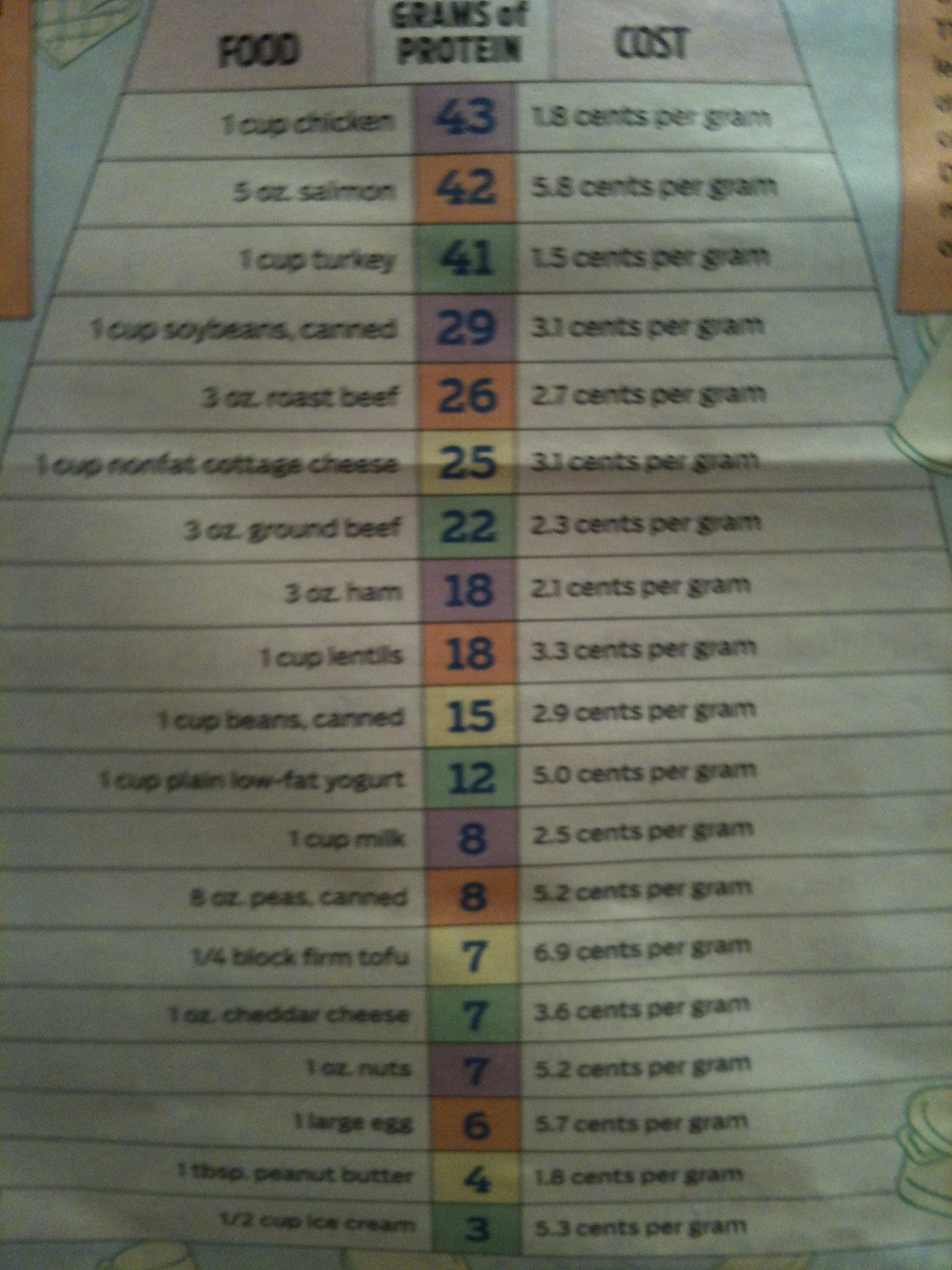The photograph depicts a color image of a chart printed on a piece of paper from a spiral-bound notebook, evident from the visible spiral binding peeking out from the top-right edge of the image. The chart is titled "Food, Grams of Protein, and Cost Chart," and it details various types of food items along with their corresponding protein content and cost per gram of protein. Although portions on the right and left edges of the chart are cut off, the primary information remains legible.

The chart is divided into three columns: 
1. **Food Type**
2. **Grams of Protein**
3. **Cost per Gram**

In the first row, for instance, "Cup of Chicken" is listed with a protein content of 4.3 grams, highlighted in a distinct second color, and the cost is indicated as 1.6 cents per gram. The background colors of the cells in the protein column vary, including shades of purple behind the protein numbers, while some entries have orange, green, or yellow backgrounds, though these colors do not follow any specific order.

Overall, the detailed chart uses a combination of textual and visual elements to convey nutritional and economical information about different protein sources, making the data easily comparable at a glance.